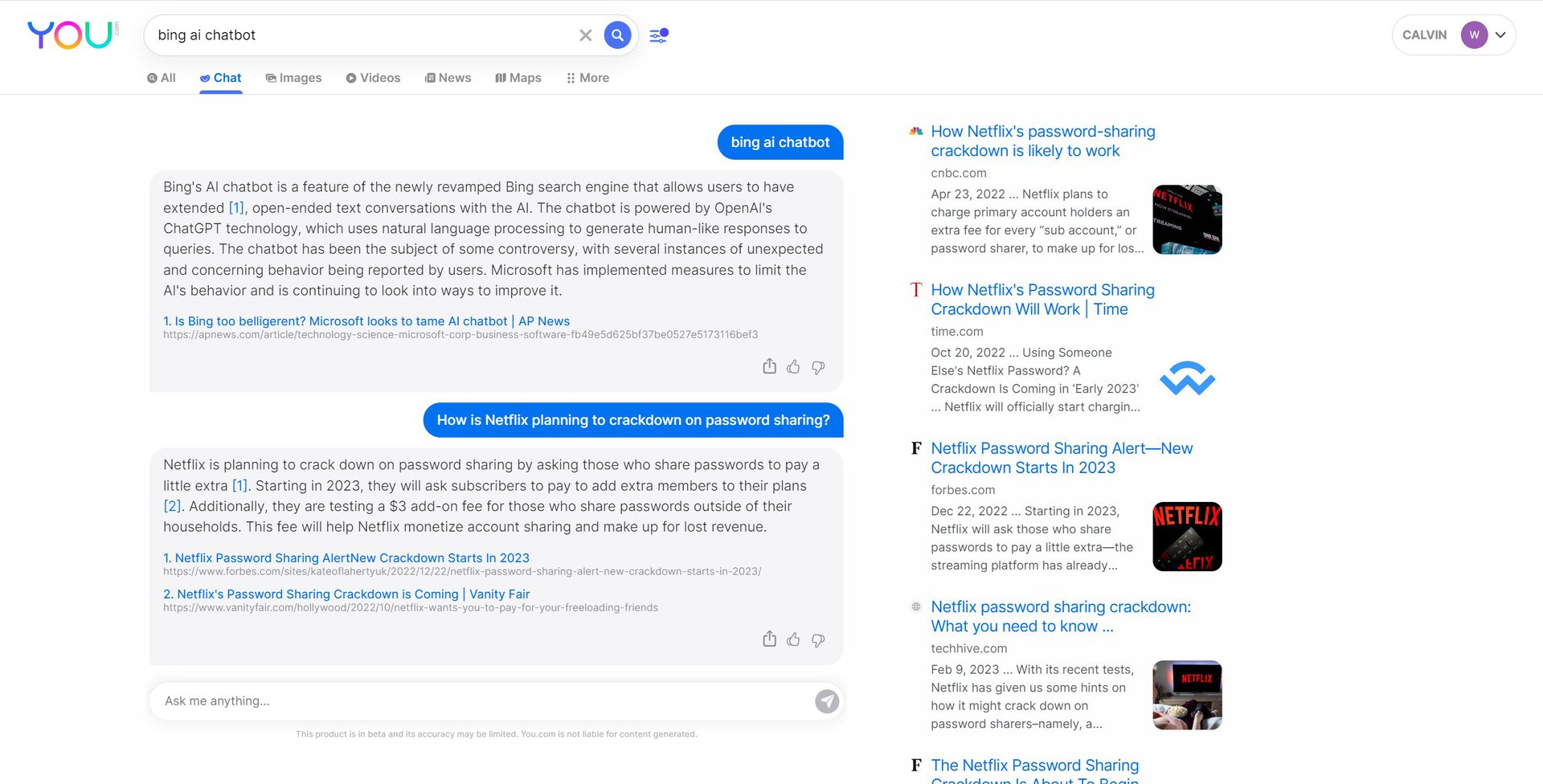This image is a screenshot of a web browser displaying a conversation on Bing AI Chatbot. At the top left, the word "YOU" is prominently written in a rainbow gradient, featuring colors blue, purple, orange, green, and blue again. In the search bar, "Bing AI chatbot" is entered, accompanied by an 'X' icon and a magnifying glass symbol. Below the search bar are clickable category links labeled: All, Chat, Images, Videos, News, Maps, and More. The 'Chat' link is currently highlighted in blue, indicating the active page.

Beneath these links, the chat interface shows an interaction. The user's query "Bing AI chatbot" appears in a blue text box, followed by a comprehensive response from the chatbot in a gray text box. In the top right corner, the user’s name "CALYN" is displayed in gray next to a purple circle with a downward arrow, implying a menu for switching users. At the bottom right, several news articles related to Netflix are visible.

This detailed description captures the layout and elements of the browser's interface, focusing on the Bing AI chat session and the surrounding features.